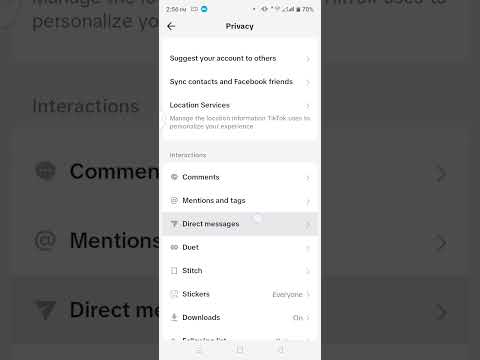This screenshot appears to be taken from a mobile device. The left and right sides of the image have been blacked out, creating a dark border. The content in the background is partially visible, displaying the word "Personalized" in the upper left, followed by the word "Interactions". Further down, fragmented text appears, showing portions of words like "common" (spelled incorrectly as "comnen") and "mentions". The word "direct" is also visible along with the letter "M", all in dark text.

In the central part of the screenshot, there is a section with a gray background and black text. At the top, the time "2:50 PM" is displayed along with two indistinct symbols. On the right side, there are various symbols that are difficult to discern. Below this, standard mobile status indicators are present, including the signal strength, Wi-Fi signal, battery icon, and battery percentage marked at 70%.

Continuing downward, the left side shows an arrow pointing left. Centered on this line is the label "Privacy". The background then transitions to a lighter color where a vertical list of gray buttons, containing options that can be clicked. These options include "Suggest your account to others", "Sync contacts and Facebook friends", and "Location services". The text "Manage the location" is visible but hard to read due to its gray color.

Below this, in black text, there is a list of interaction categories which include "Comments", "Mentions and tags", "Direct messages", "Duet", "Stitch", "Stickers", and "Downloads". This detailed information concludes the visible part of the screenshot.